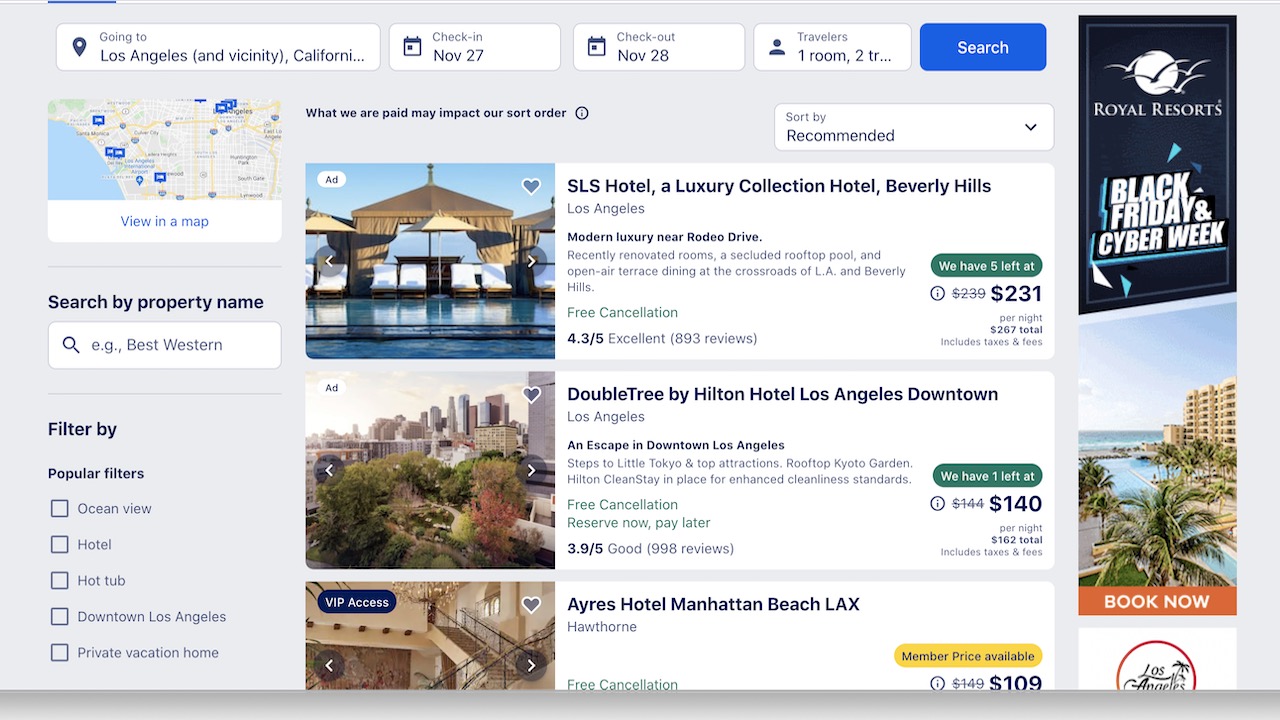A screenshot of a travel website's interface is depicted, revealing various search and filter functionalities. At the very top, a navigation bar includes several input fields: a destination box labeled "Going to," a "Check-in" date box, a "Check-out" date box, a box indicating the number of travelers, and a "One room" selection. To the right of these fields, a prominent blue search button is visible.

Directly below, on the left side of the screen, there is a map with an option to "View in a map" displayed beneath it. On the right, a search bar labeled "Search by property name" provides additional search functionality. Adjacent to this, there is a "Filter by" section featuring "Popular filters" with various checkboxes for different filtering options.

Further to the right, black text indicates "Sort order." Below this, a white dropdown box labeled "Sort by Recommended" allows users to sort search results. The main content area features three hotel options, each within its own box. Every box comprises a hotel image on the left and, on the right, the hotel's name, a brief description, and the price noted in the bottom-right corner.

On the far right side of the screen, several advertisements are present. One promotes Royal Resorts' Black Friday and Cyber Week deals, another encourages booking now for an unspecified hotel, and a partial ad features a circular logo with the text "Los Angeles."